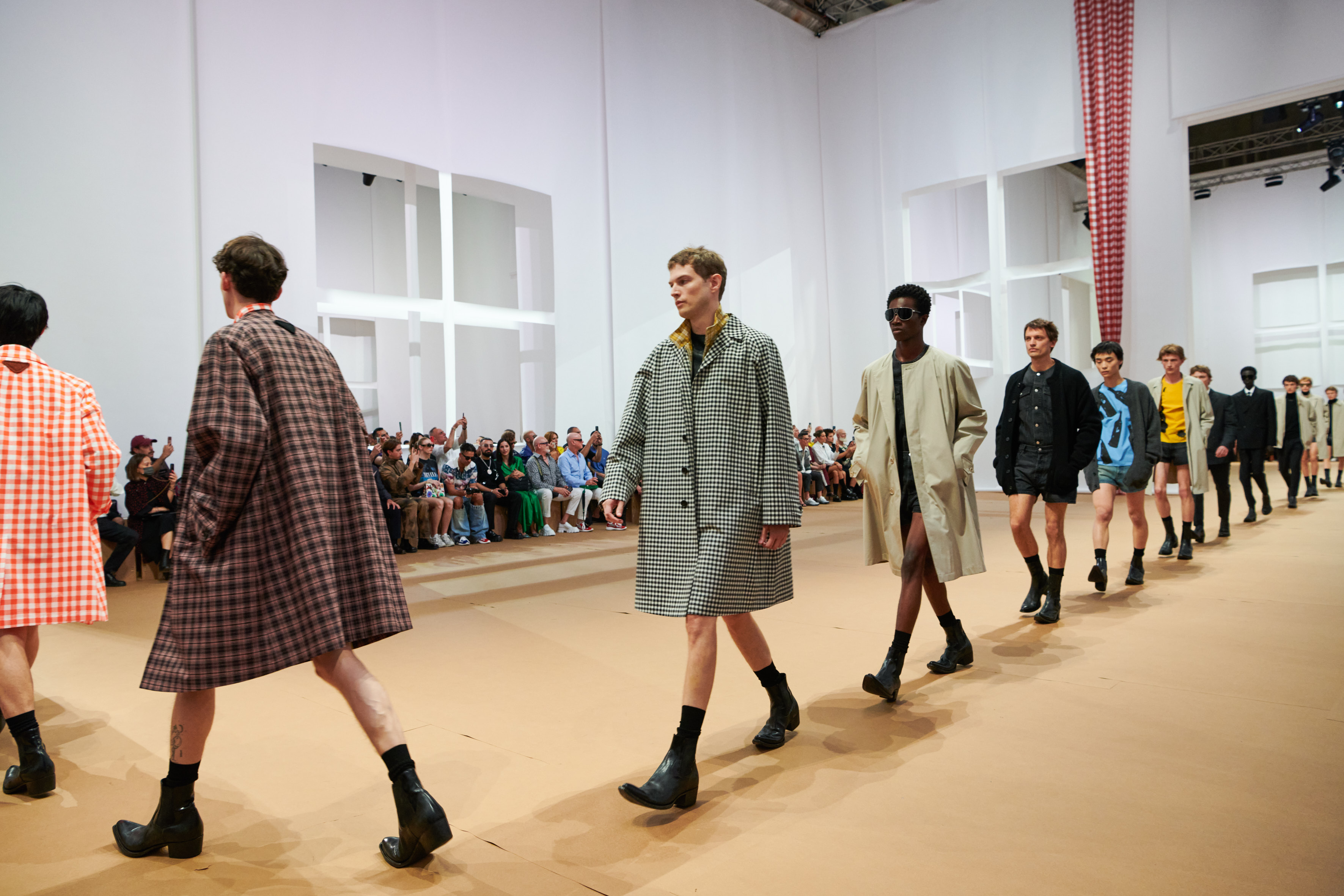This color photograph in landscape orientation captures an interior scene of the Prada fashion show, featuring a line of male models on a cream-colored catwalk with white walls in the background. The models, ranging in various sizes, colors, and ages, are mostly seen wearing knee-length plaid checkered coats in different hues, paired with dark boots and socks. Some models appear to have shorts underneath their coats, though not entirely visible. The lineup begins at the center-right of the image, proceeding toward the bottom left corner, where the lead model turns and continues to the left. The closest model to the viewer, positioned in the bottom left with his back facing outward, sports a beige and black checked coat, while the next visible model dons an orange and white checked coat. A crowd of spectators is seated and taking pictures on the left side of the runway against the backdrop of large cross-shaped windows. Studio lights illuminate the scene, and in the distance, a red and white checkered curtain hangs, accentuating the spacious, open atmosphere of the venue.